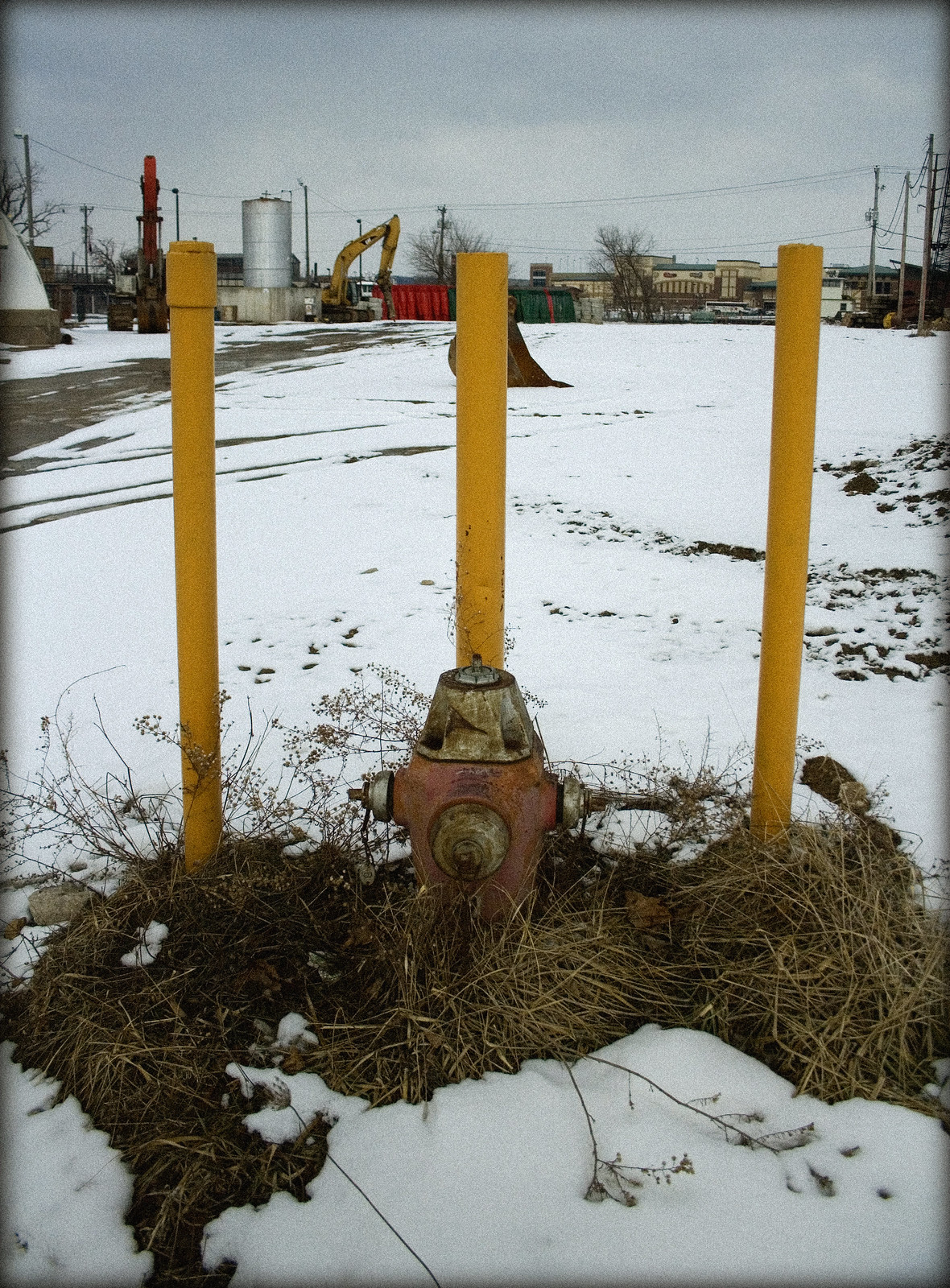In this photograph, an old, weathered fire hydrant stands prominently in the bottom middle of the scene. Once red, the hydrant now bears a faded pink hue with patches of rust near the top. It sits in a clump of dry, brown grass amidst a snowy landscape. Surrounding the hydrant are three tall, yellow posts, approximately 3-4 feet high, one of which is topped with a matching yellow cap, presumably to protect the hydrant from vehicular impact. 

In the background, across a lightly dusted snowy field marked by tire tracks, various construction machinery is visible, including diggers, cranes, and a distant steam shovel bucket behind the middle post. A dirt path, worn down by traffic, extends to the upper left of the image. Along the horizon, a building with a metal silo stands, accompanied by a large device with a red protruding part, and a cluster of large buildings possibly belonging to shopping centers. The sky above is gray and cloudy, casting a muted light over the scene. Despite the snow, details of a bustling industrial and urban area can be discerned in the distance.